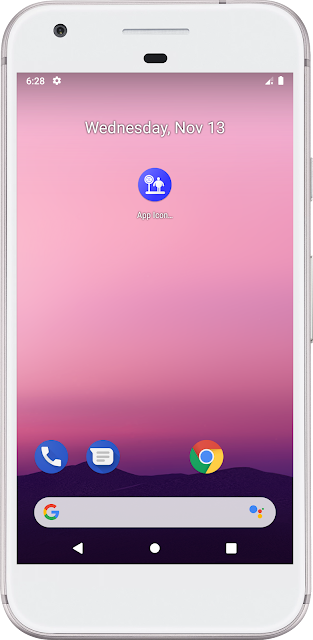This image is a detailed close-up of an Apple mobile phone, showcasing both the device and its screen. The phone has a white case and features the power and volume buttons on the right edge. At the top left corner, a camera lens is visible.

The phone's screen displays a beautiful pink and purple landscape wallpaper, depicting the top of a hill under a vibrant sky. The status bar at the very top shows the time as 6:28 AM. To the right of the time, there's a gear icon, and on the far right, a fully charged battery icon is displayed.

The date and day "Wednesday, November 13th" are prominently featured on the home screen. Below this, there's a blue icon with a silhouette of a person standing next to what appears to be a fan, labeled as "App Icon." At the bottom of the screen, three icons are neatly lined up: a blue call button on the left, a messaging app button in the center, and a Chrome browser icon on the right. Below these icons, a Google search bar is visible.

The overall design is clean and user-friendly, highlighting the phone's functionality and aesthetic appeal.